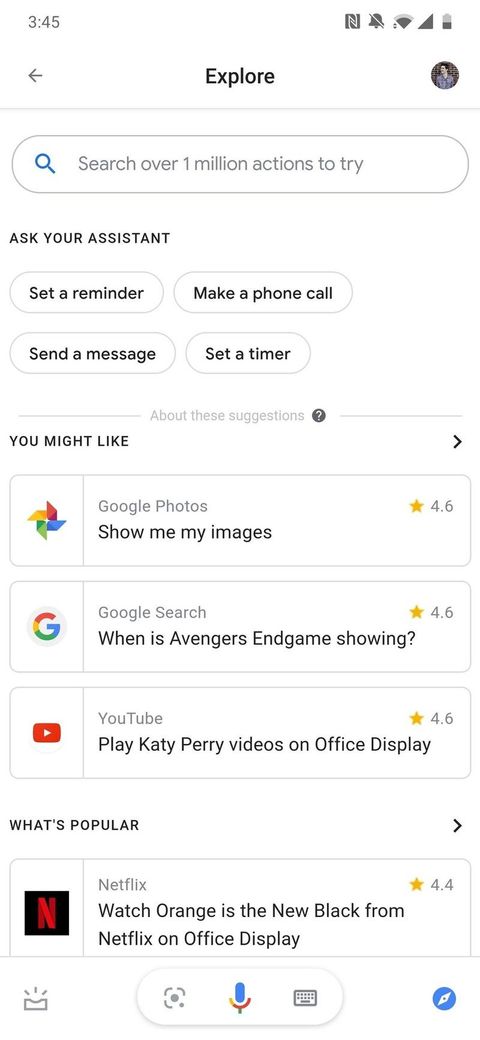Screenshot of a digital assistant interface showcasing various functionalities and suggestions

At the top of the screen, the status bar displays the time, 3:45 PM, alongside several icons, including a near-field communication (NFC) symbol, a muted notifications bell, a Wi-Fi signal indicator, and a battery icon. Below the status bar, a back arrow appears next to the word "Explore" in black text. Adjacent to this is a circular profile picture placeholder, followed by a gray search box accompanied by a blue magnifying glass icon and the text, "Search over 1 million actions to try."

Moving down the interface, four interactive suggestion boxes are present under the heading "Ask your assistant." These boxes offer quick access to actions like "Set a reminder," "Make a phone call," "Send a message," and "Set a timer." Further down, a section titled "About these suggestions" marked with a question mark provides additional context or information.

The screen continues with a "You might like" section featuring recommended apps and actions. The first recommendation is "Google Photos," identified by its distinctive multicolored icon (gold, red, green, and blue) and rated 4.6 stars with a gold star. Below it is the "Google Search" app, also displaying a multicolored (red, gold, green, and blue) icon and rated 4.6 stars, with a sample query: "When is Avengers Endgame showing?". The "YouTube" recommendation follows, symbolized by the red and white play button and suggesting the action: "Play Katy Perry videos on Office Display," rated 4.6 stars as well.

The interface also highlights a "What's popular" section featuring the "Netflix" app. The Netflix icon is black and red, and the recommendation is to "Watch Orange is the New Black from Netflix on Office Display," which is rated 4.4 stars, signified by a gold star.

At the bottom of the screen, a variety of icons can be seen, including a box with wavy lines, a square, a multicolored (blue, gold, and red) microphone icon, a gray keyboard, and a blue circle with a white mark in its center.

This detailed screenshot captures the diverse features and suggestions offered by the digital assistant interface.